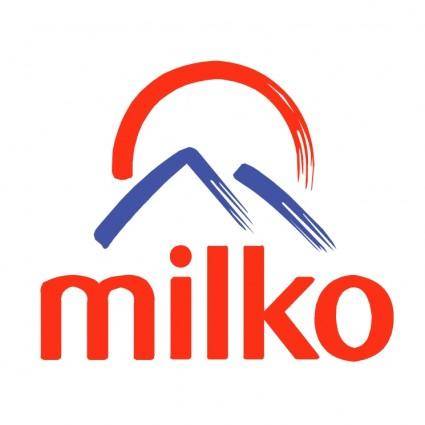The image features a company logo set against a white background. Dominating the lower portion of the image is the brand name "Milko" displayed in red, lowercase letters, M-I-L-K-O. Above the letters, there is abstract imagery reminiscent of a mountainous landscape composed of two blue, paintbrush-like slashes. The first blue streak forms a greater-than sign with its tip pointing downwards, while the second blue streak sits beside it, creating the illusion of two mountain peaks. A red semicircle, also appearing as a paintbrush stroke and feathered at the bottom, arches above the blue mountains, symbolizing a rising sun. The design employs a loose, artistic style with just two colors: blue for the mountains and red for both the text and the sun, creating a visually striking contrast against the white background.